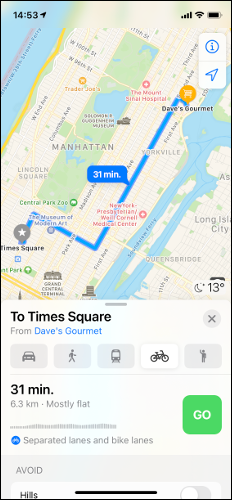This image is a snapshot of a navigational map showing the cycling route from Times Square to Dave's Gourmet. 

Prominently featured in the center of the map is a blue line representing the 31-minute bike route between the two locations. The map spans a portion of Manhattan and includes notable landmarks such as Queensbridge, Yorkville, and Mount Sinai Hospital. The screen displays the current time in military format, showing 14:53 (2:53 PM), and indicates favorable conditions for electronic device usage, with a high battery level and a robust internet connection. 

The interface also provides crucial trip details: a temperature of 13 degrees Celsius, and specific data points about the bike route—indicating it covers a distance of 6.3 kilometers, is mostly flat, and includes both separated and dedicated bike lanes. Users see various travel options at the bottom, with the bike option highlighted, featuring a green "GO" button in white letters for easy commencement of the journey. There's also an "Avoid" option on the left, allowing the user to steer clear of hilly terrains by toggling a designated button.